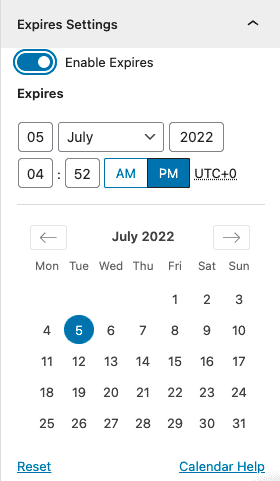The screenshot captures an interface for managing expiration settings on a website. At the top, there's a light gray banner that reads "Expires Settings" with an upward arrow icon, denoting navigation or adjustment ability. Below the banner, a white background features a circular toggle switch, currently set to the right to indicate that the "Enable Expires" option is activated. The word "Expires" is labeled beneath the toggle.

Further down, a series of dropdown menus and input fields are displayed to set specific expiration dates and times. A small square field shows "05" next to another dropdown labeled "July," followed by a square field for the year "2022." 

Beneath this row, time settings are presented: a square field reads "04" for hours and another with "52" for minutes. Time of day is set with AM/PM selectors, and PM is currently selected. The time zone is displayed as "UTC +0". 

A dotted line separates this section from the calendar widget below. The calendar displays navigation buttons with left and right arrows, flanking the label "July 2022" at the top. The days of the week are abbreviated to three letters each, starting from Monday to Sunday. Corresponding dates for the days fall directly below.

At the bottom, buttons labeled "Reset," "Calendar," and "Help" offer additional options to manage and configure settings.